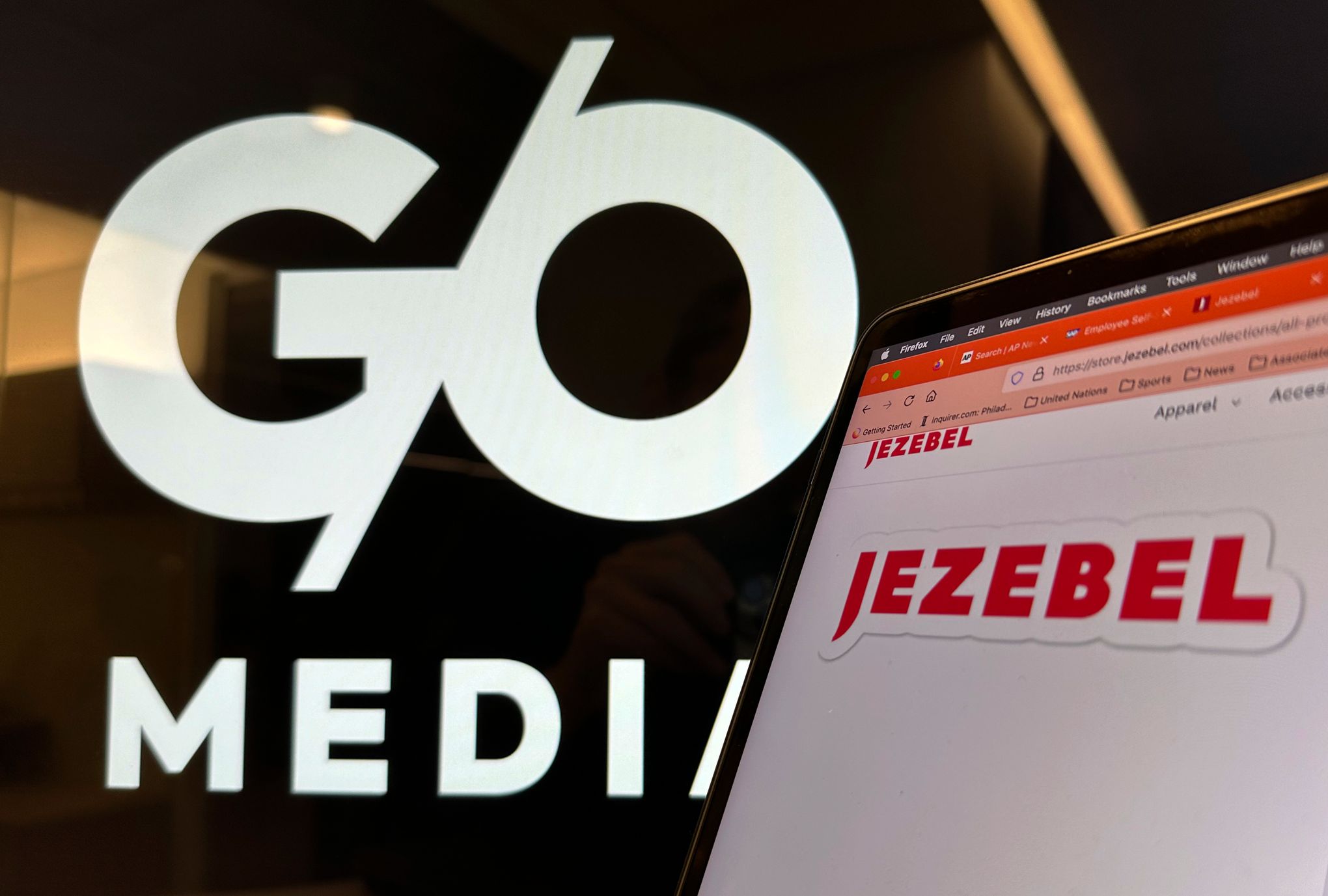This image appears to be a detailed advertisement for a media company. On the left side, it prominently displays the text "G/O" in large white font on a black background, followed by the smaller, capitalized letters "MEDI". The right side of the image features a partial, three-quarter view of an Apple laptop screen, with the small white Apple logo visible, indicating it's a Mac. 

The laptop screen shows a white webpage from a website called Jezebel, prominently featuring the dark red word "Jezebel" in the top left corner. Below this, the webpage lists categories such as "Apparel" and "Accessories," suggesting that Jezebel is an e-commerce site. An orange taskbar is also visible on the browser, and along the top of the monitor are options including view, history, bookmarks, and tools, indicating it is a typical web browser interface. A subtle hand is seen holding the laptop or taking a picture of the scene. 

The image combines the branding of both the media company, G/O Media, and the website, Jezebel, with the distinct black and white contrasted background and the clear depiction of the Jezebel website on the laptop screen.